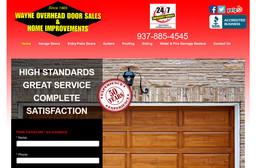This image seems to be an online advertisement for Wayne's Overhead Door Sales and Home Improvements. It prominently features the company's logo and name at the top, with a clear emphasis on service hours, showcasing a 24/7 availability notice. Adjacent to the 24/7 logo is the Better Business Bureau accredited symbol, reinforcing the company's credibility.

In the top right corner, the advertisement displays various social media icons, including Facebook and Twitter, allowing customers to connect with the company via multiple platforms. Beneath these social icons, there is a section likely dedicated to product support and contact information, although some text is unclear.

Central to the advertisement is a high-quality image of a garage door, illustrating the type of products offered by Wayne's Overhead Door Sales. To the left of this image, in white text on a black background, the company highlights its commitment to "High Standards, Great Service, Complete Satisfaction."

At the bottom of the ad, there is a form where potential customers can enter their email and contact information to receive updates, deals, and coupons.

Overall, the advertisement effectively markets Wayne's Overhead Door Sales and Home Improvements, combining visual elements with key information to attract and inform potential customers.